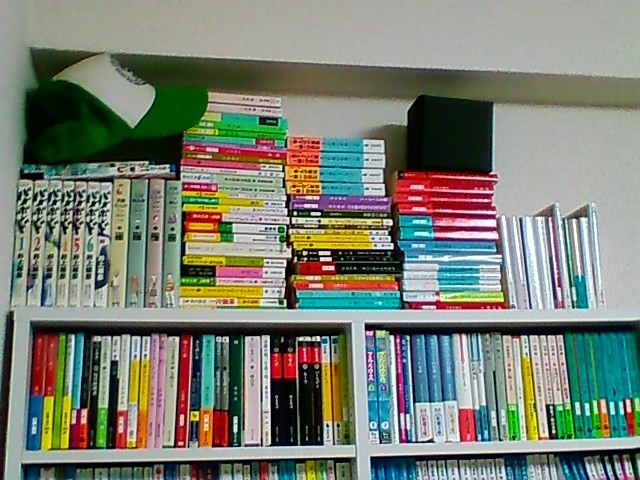This color photograph showcases a packed bookshelf nestled in a small alcove of a white wall, with books filling the visible three shelves entirely. The books vary in width, height, and color, and many seem to be educational. The top shelf overflows with vertically standing books, further topped by horizontally stacked ones, extending almost to the ceiling. On the far top left, a green and white baseball cap with a green logo is tucked among the books. Among the diverse collection, there is a distinctive series, possibly manga, positioned on the bottom and left levels. This series, featuring numbers 1 through 6 or 7, appears to be written in either Mandarin or Japanese kanji. The overall organization reflects a personal collection, not a library, given the absence of categorization labels.